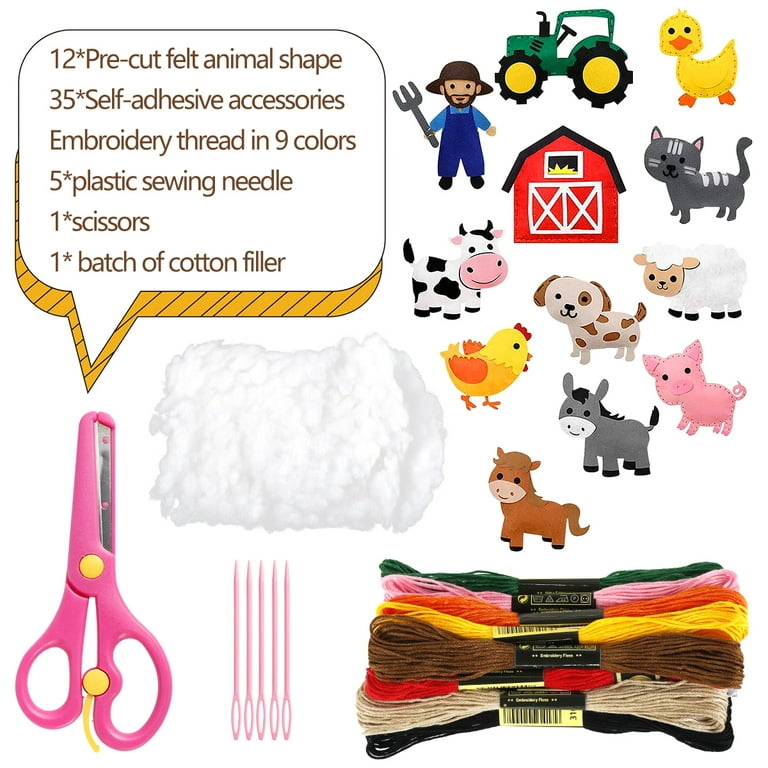The image depicts a comprehensive craft set. On the left side, there's a detailed text box listing the contents: 12 pre-cut felt animal shapes, 35 self-adhesive accessories, embroidery thread in nine colors, five plastic sewing needles, one pair of pink scissors, and one batch of cotton filler. The pink scissors and needles are prominently placed on the left. The center left features a batch of white cotton filler. The right side showcases cartoon depictions of various farm animals and related images, including a green tractor, a farmer, a barn, a duck, a cat, a cow, a sheep, a dog, a chicken, a pig, a donkey, and a horse. Below these illustrations, bundles of embroidery thread in diverse colors such as green, pink, orange, yellow, brown, red, beige, and black are displayed.